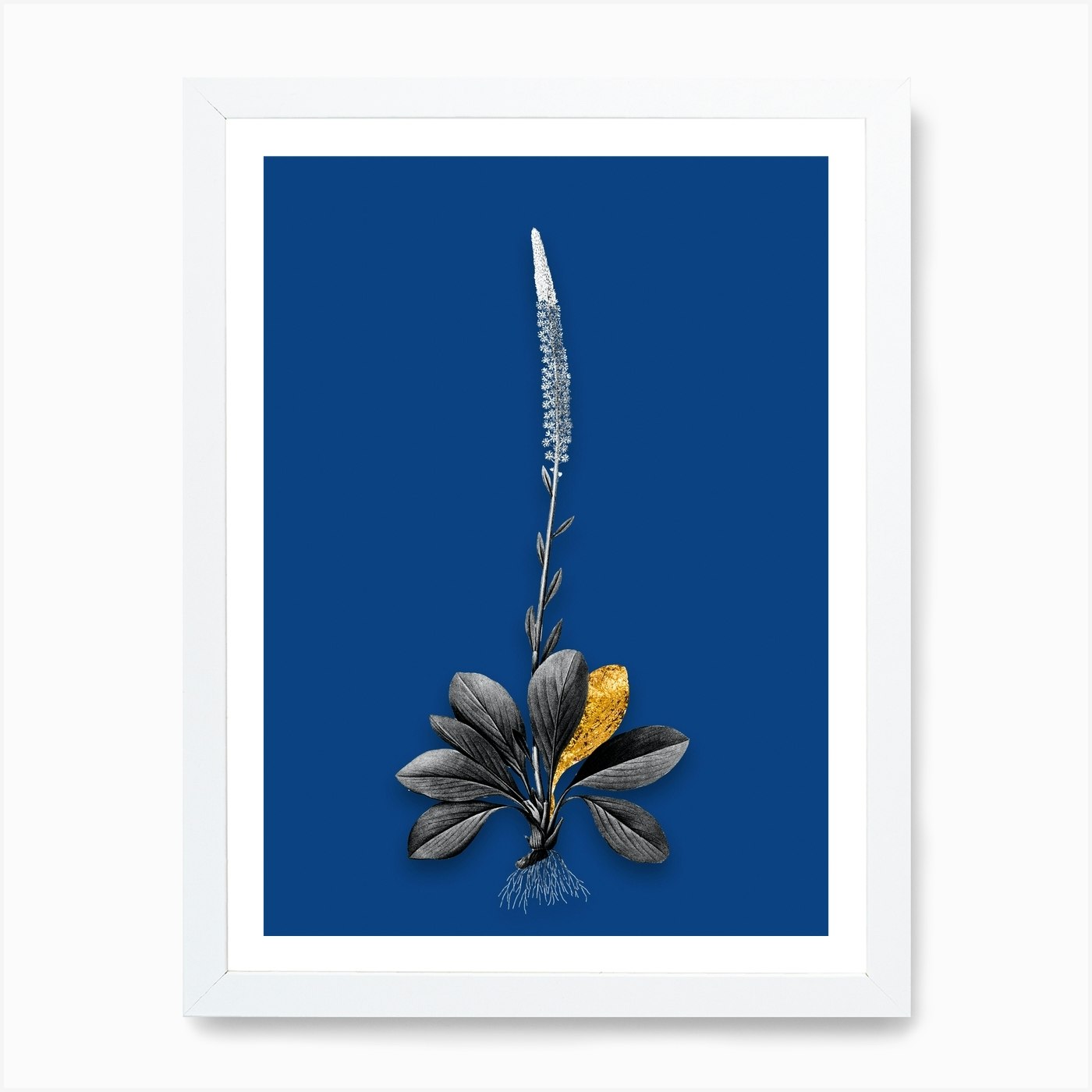This is a detailed illustration of a plant, meticulously pressed onto a deep blue background and framed with a light blue outer border and a crisp white inner border. The picture frame hangs on a white wall. The plant appears to have been pulled out of the ground, with its small roots, which are light blue, visible at the base. From the roots, a main stem extends upward for about eight inches. Surrounding the base of the stem are several leaves, fanning out like a deck of cards. Most of the leaves are black, except for one vibrant gold leaf that stands out prominently. The stem is adorned with tiny, delicate leaves that continue up each side. As it approaches the top of the frame, the stem features minuscule white flowers that intensify in density, culminating in a solid white tip. The overall appearance is that of a plant carefully preserved in its entirety and showcased in an elegant, minimalist frame.